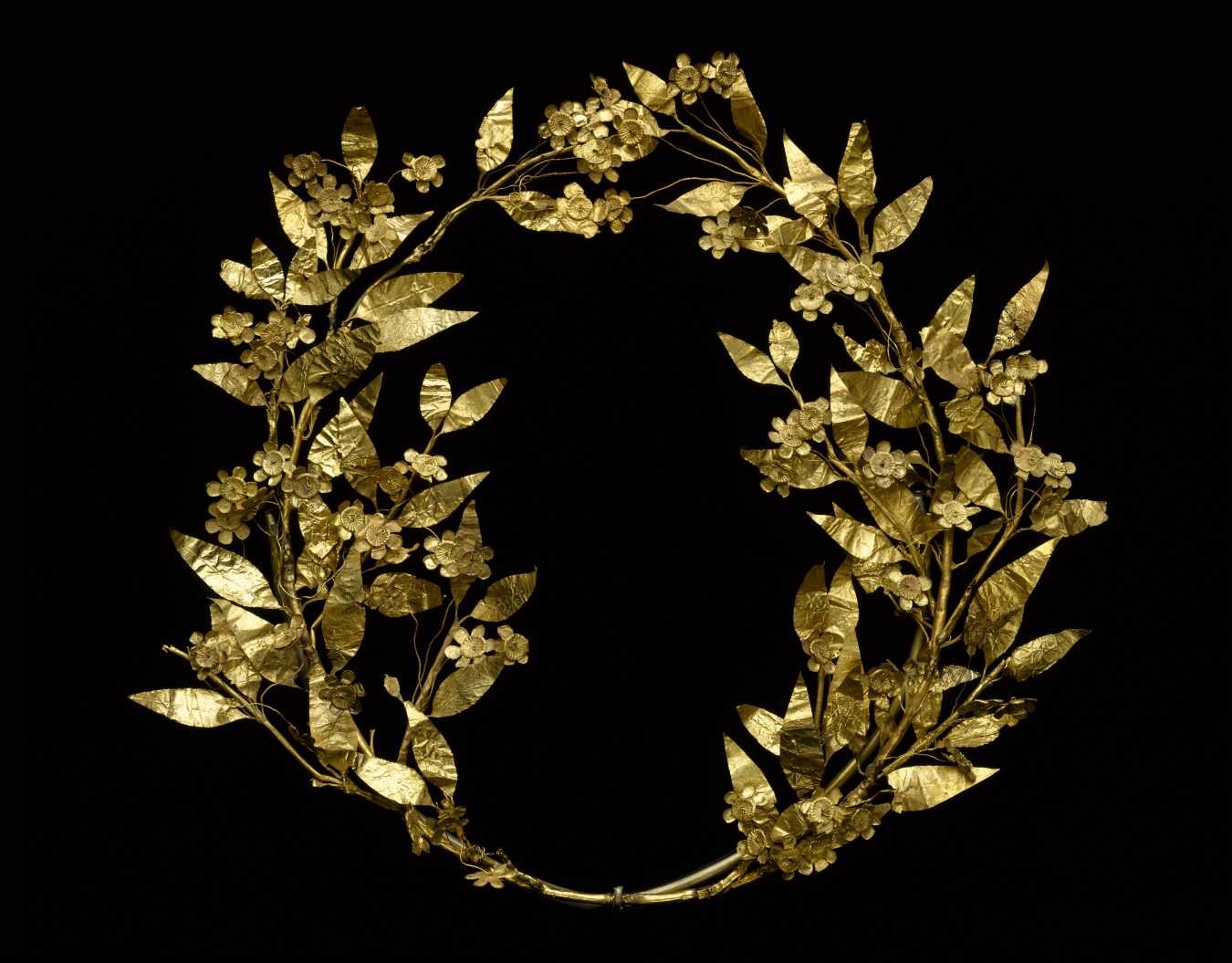The image depicts a meticulously arranged, high-quality studio-like photograph of golden, leafy branches intricately shaped into a circular wreath. Set against a giant, stark black background, the wreath exudes a sense of antiquity and opulence. It's composed of two winding branches, adorned with golden leaves and small blossoming flowers, that start intertwined at the bottom and rise gracefully to meet again at a single point at the top. This formation gives it an imperfect, yet elegantly natural circular form. The wreath possesses an air of regal craftsmanship, reminiscent of artifacts worn by royalty in ancient Greece or Rome, and it seems almost ready to be placed decoratively or worn as a crown. The lighting enhances its intricate details, making it appear almost luminous against the dark backdrop.